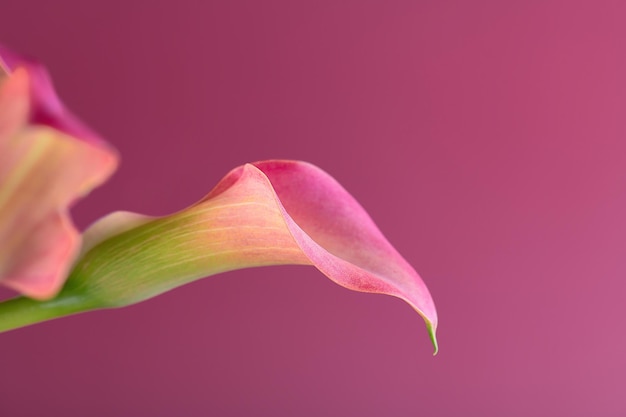This image depicts what appears to be a painting on canvas, dominated by shades of pink. At the center, emerging from the left side, are two flowers. The main flower, which is most likely an orchid or possibly a Kala lily, stands partially bloomed with its petals yet to fully unfurl, displaying a mix of pink with hints of green and a touch of yellow. The lower portion of this flower transitions to a light green, matching its single visible green stem. Another blurred bloom of a similar hue is seen in the background, adding depth to the composition. The dark pink background gradually lightens from one side to the other, creating a harmonious blend that makes the flowers partially merge with the canvas, enhancing the painterly effect.